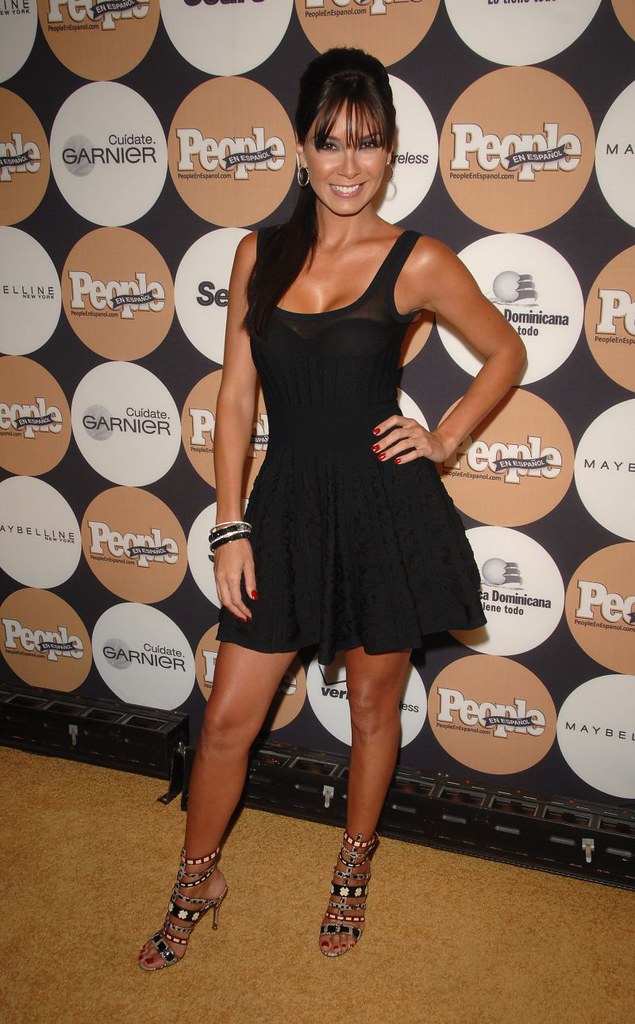A tanned woman, who appears to be a celebrity, is posing at an event on a gold-colored carpet. She has brown hair styled in a high ponytail with long bangs framing her face. She is smiling broadly and showcasing red fingernail polish. She is dressed in a chic black dress that reaches her mid-thigh, revealing her bare legs, and accessorized with black and silver bracelets on one wrist. Her high-heeled sandals have multiple colorful straps. The woman is striking a confident pose with her left hand on her hip. Behind her is a backdrop adorned with beige and white circles advertising various brands, including "People en Español," "Ciudád Garnier," "Maybelline," and "Dominicana." The display conveys an array of product promotions, highlighting Garnier's logo prominently.